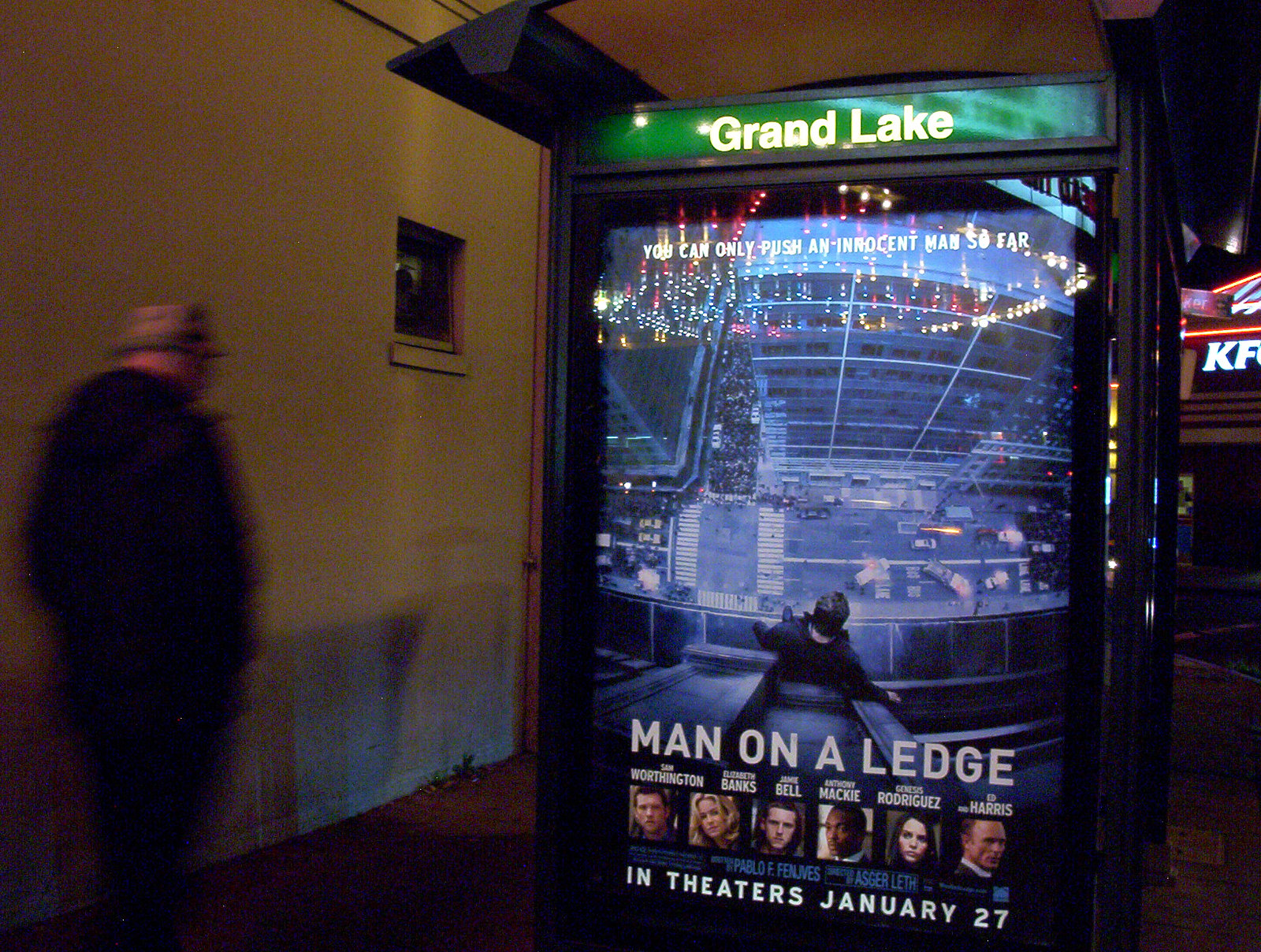In the image, we see a dimly lit setting, possibly a mall or food court, with a carpeted floor and a wall on the left side. The wall features a small window, and a man dressed in a black jacket, pants, and a hat is walking away from the camera. Central to the image is a prominently displayed digital sign that reads "Grand Lake," with vibrant colors including green, tan, black, pink, gray, orange, yellow, and purple. Beneath this, there is a digital movie poster for the film "Man on a Ledge," depicting a man standing on the edge of a building and looking down. The caption reads, "You can only push an innocent man so far." The poster lists the cast, including Sam Worthington, Elizabeth Banks, Jamie Bell, Anthony Mackie, Genesis Rodriguez, and Ed Harris. It also notes the release date, "In theaters January 27th." The setting includes reflections from overhead lights on the glass encasing the poster. In the distance to the right, there's a partially visible sign for a KFC restaurant. A blurry image of the man walking near the wall adds to the bustling atmosphere of this urban interior scene.